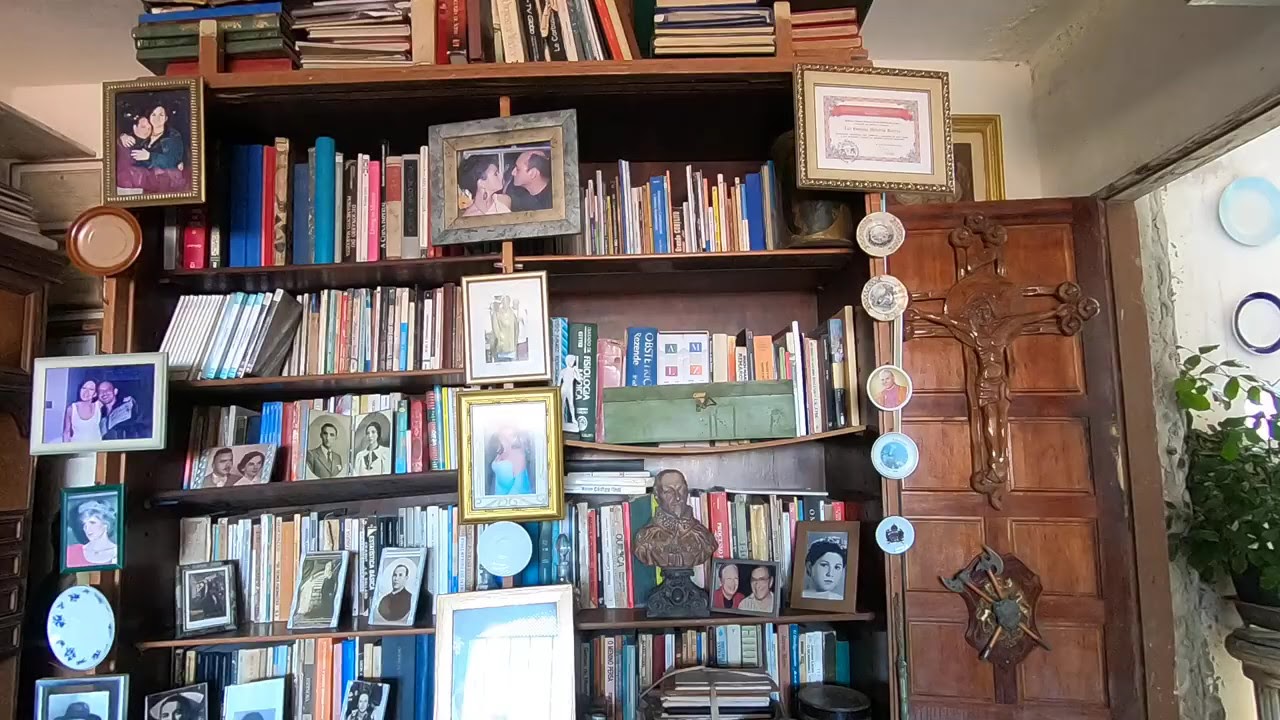The image depicts a large, ornate wooden bookcase, most likely crafted from cherry wood, standing inside someone's home. The bookcase has four shelves packed with various books, though their titles are not readable. Scattered among the books are multiple framed family photos, including an old black-and-white picture of a couple kissing, possibly the homeowner's parents or grandparents, and an image of a person wearing a tiara. Centered among the photos is a framed diploma, flanked by several displayed buttons beneath it. 

A notable feature on the bookcase door is an intricate carving of Jesus on the cross, measuring approximately two feet long by 18 inches wide, emphasizing its Catholic iconography. Below the cross is an ornate shield displaying two medieval battle axes, suggesting a family crest. Additionally, on the second shelf to the right, there is a bust of a man. Prominently set against the bookcase's upper sections are more family photos interspersed with decorative items like small plates. To the far right, outside the bookcase, part of the house's white wall and a houseplant are visible, adding to the image's domestic setting.